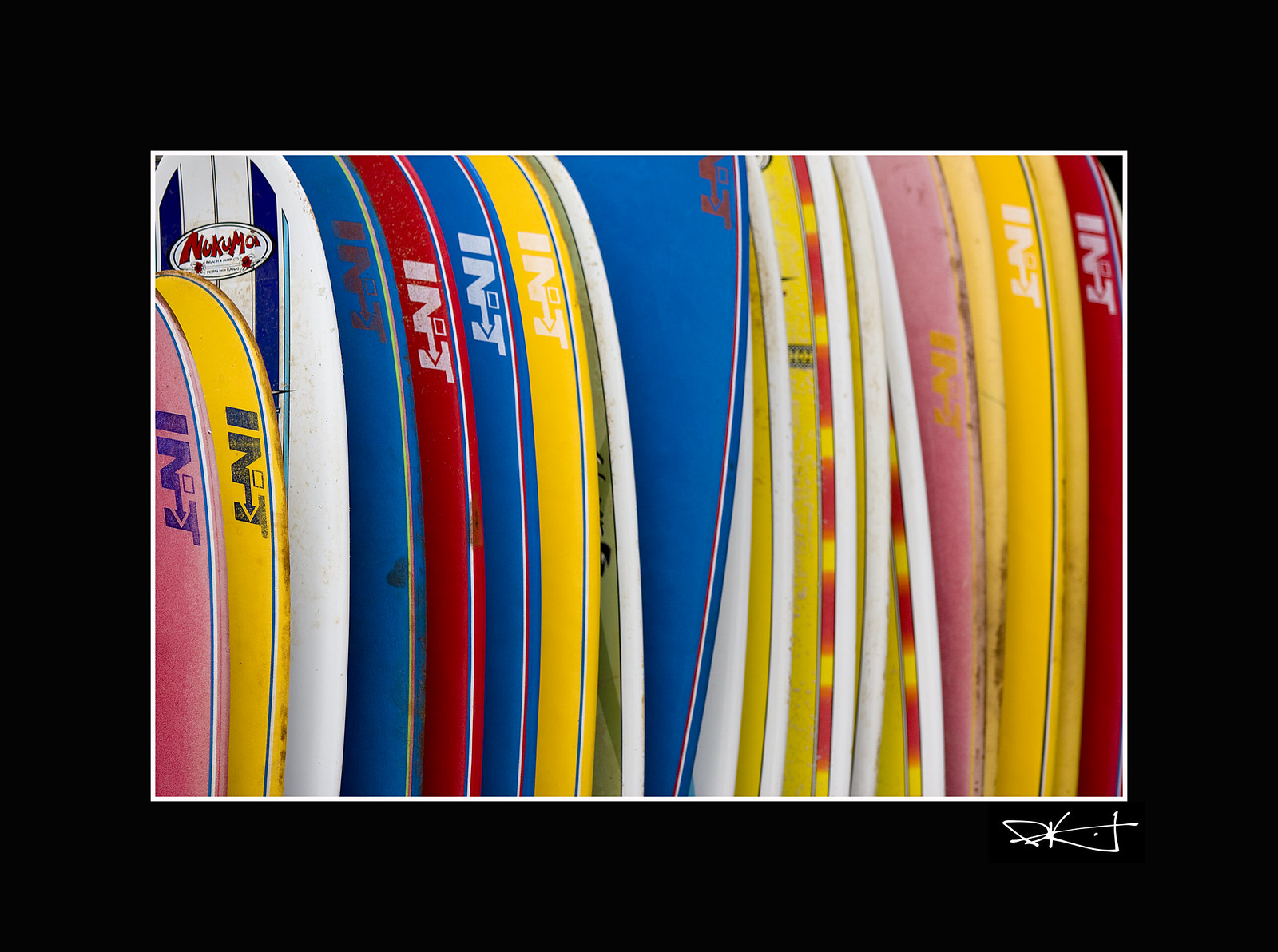This horizontal photograph, well-lit and bordered by a thick black mat, showcases a close-up view of various surfboards and body boards standing vertically. The boards are depicted in a variety of vibrant colors, including red, blue, white, yellow, and pink, often adorned with alternating color patterns. Each board features the initials "INT," with the "N" forming an arrow pointing into the "T." The black border surrounding the photograph includes a script signature in the lower right-hand corner, ending in the letter "T" and potentially indicating the artist's initials as "RK." The composition of the boards, partially visible in the narrow, zoomed-in shot, resembles stacked dominoes, lending an abstract aesthetic to the piece.